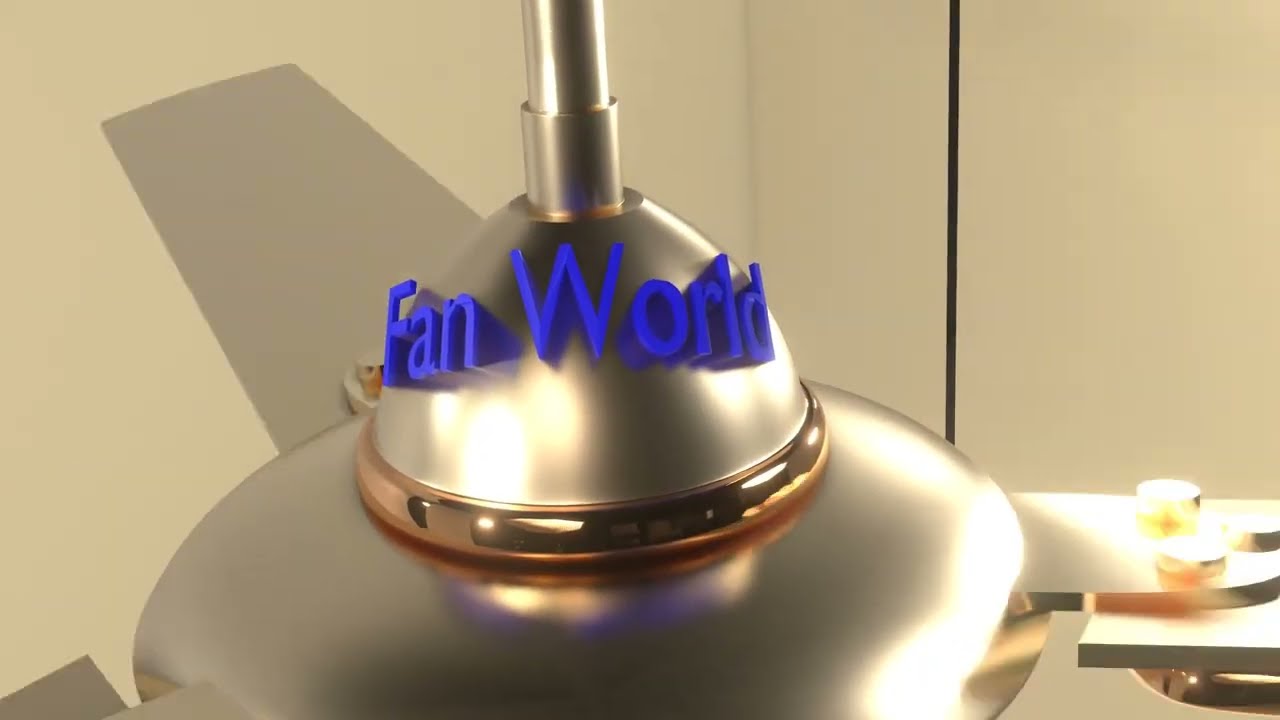The image captures a detailed, zoomed-in view of a silver ceiling fan from an elevated angle. The fan hangs from a cylindrical silver rod attached to a domed housing that contains the motor. Prominently displayed across the dome in a 3D, blue sans-serif font is the text "Fan World." The font is warped in the center and features a darker blue shadow effect. The image shows three fan blades projecting from the motor housing—one extending towards the top left, another towards the right, and the third towards the bottom left. Each blade is mounted on a circular hub with shiny gold bolts. Additionally, a black rope is visible extending from the fan housing towards the ceiling. The background consists of white walls with a light gray corner line, adding a sense of depth. The setting could be interpreted as either a home or a showroom for fans. The overall color palette includes silver, blue, white, black, light yellow, and subtle hints of gold.